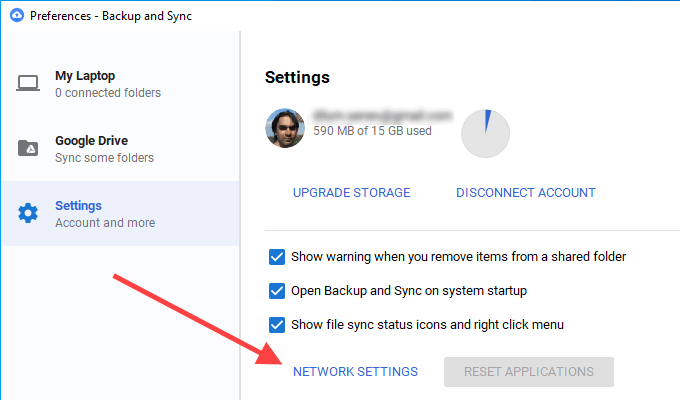The image depicts a detailed interface of a software application, likely a cloud storage service such as Google Drive's Backup and Sync utility. At the top of the interface is the title "Settings" in black font. 

The left-hand section of the interface has a vertical menu starting with "Preferences," "Dash Backup," and "Sync" in black font. Below this menu is a descriptive section showing "Black Laptop," indicating the device name, followed by "Zero Connected Folders," "Google Drive," and "Sync Some Folders." An adjacent blue gear icon is labeled "Settings" in blue text, underlined by another descriptive word in black.

A red arrow on the screen points downward from this area towards the bottom-right section of the interface. Here, there is an option labeled "Network Settings" in blue, next to a gray rectangle labeled "Reset Application." Above this section, in black text, are the options "Show Sync Locations Icons" with a right-click menu. This section is marked with a blue box containing a white checkmark. 

Higher in the interface, another two blue boxes with white checkmarks are visible. The first one reads "Open Backup and Sync on System Startup," and the second reads "Show Warning when you remove items from a shared folder." 

A thin gray line horizontally divides these sections. Above this line, two options in all capital letters and blue font are present: "Upgrade Storage" on the left and "Disconnect Account" on the right.

Additionally, there is a pie chart near the top, predominantly gray with a small blue slice, representing storage usage. The chart is annotated with "590 MB of 15 GB Used," indicating the storage utilization.